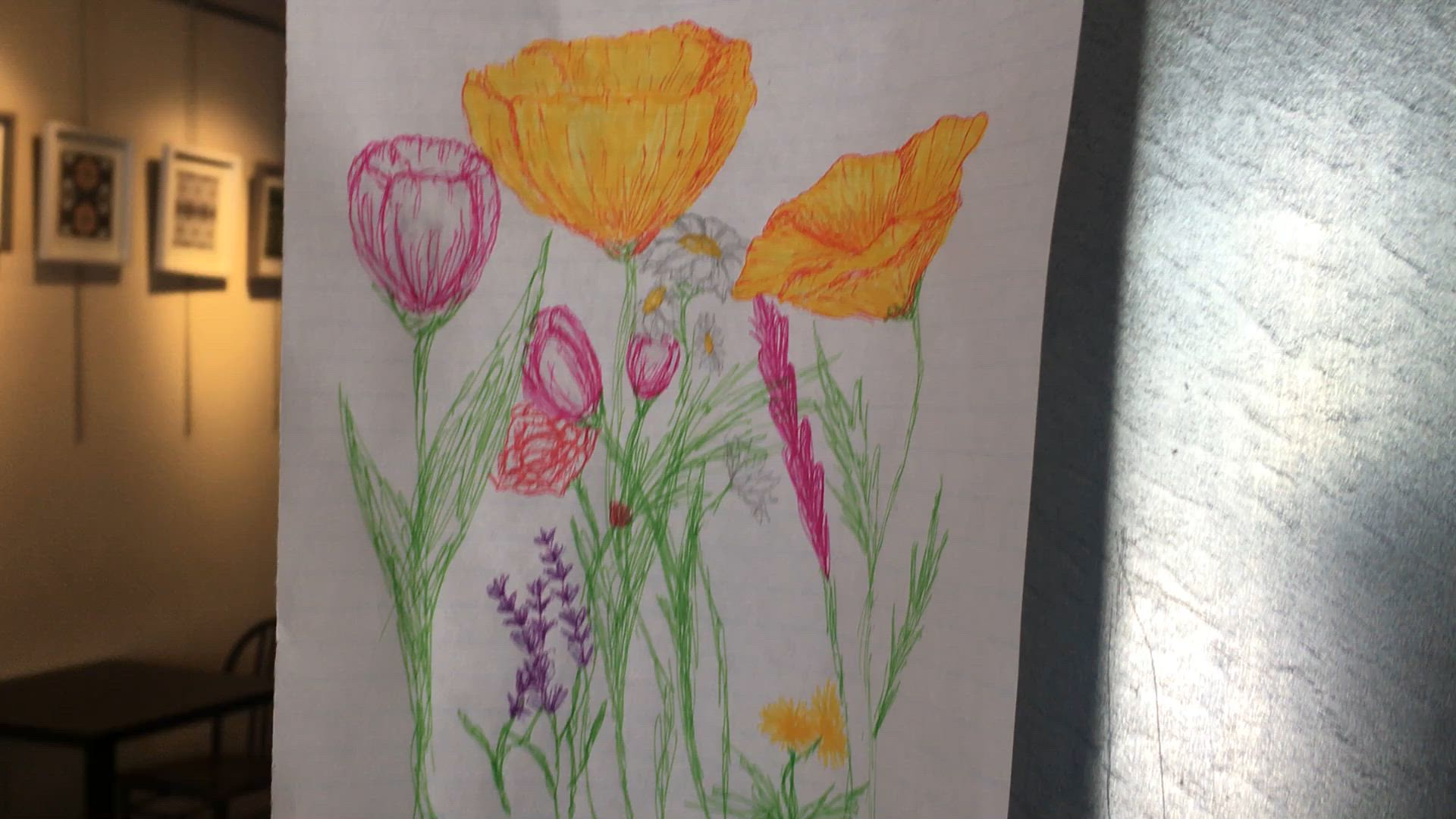This color photograph, taken inside a cozy home, reveals a charming and artistic corner of a room. On the left-hand side of the image, there are four framed pieces of artwork. Two of the frames are black, and two are white, each containing distinct pieces of art. Below these frames, there is a small table paired with a chair, adding a touch of functional decor to the space. 

Central to the photograph is a piece of notebook paper delicately displayed on the wall, mimicking the framed artworks around it. This paper is adorned with an array of vividly colored flowers, including purple and pink blossoms, a white daisy, vibrant orange and yellow tulips, and cheerful sunflowers. The flowers are a mixture of fully bloomed and budding stages, bringing a sense of life and growth to the scene. This whimsical and colorful drawing acts as an ephemeral addition to the home's curated art collection, blending creativity and everyday simplicity.